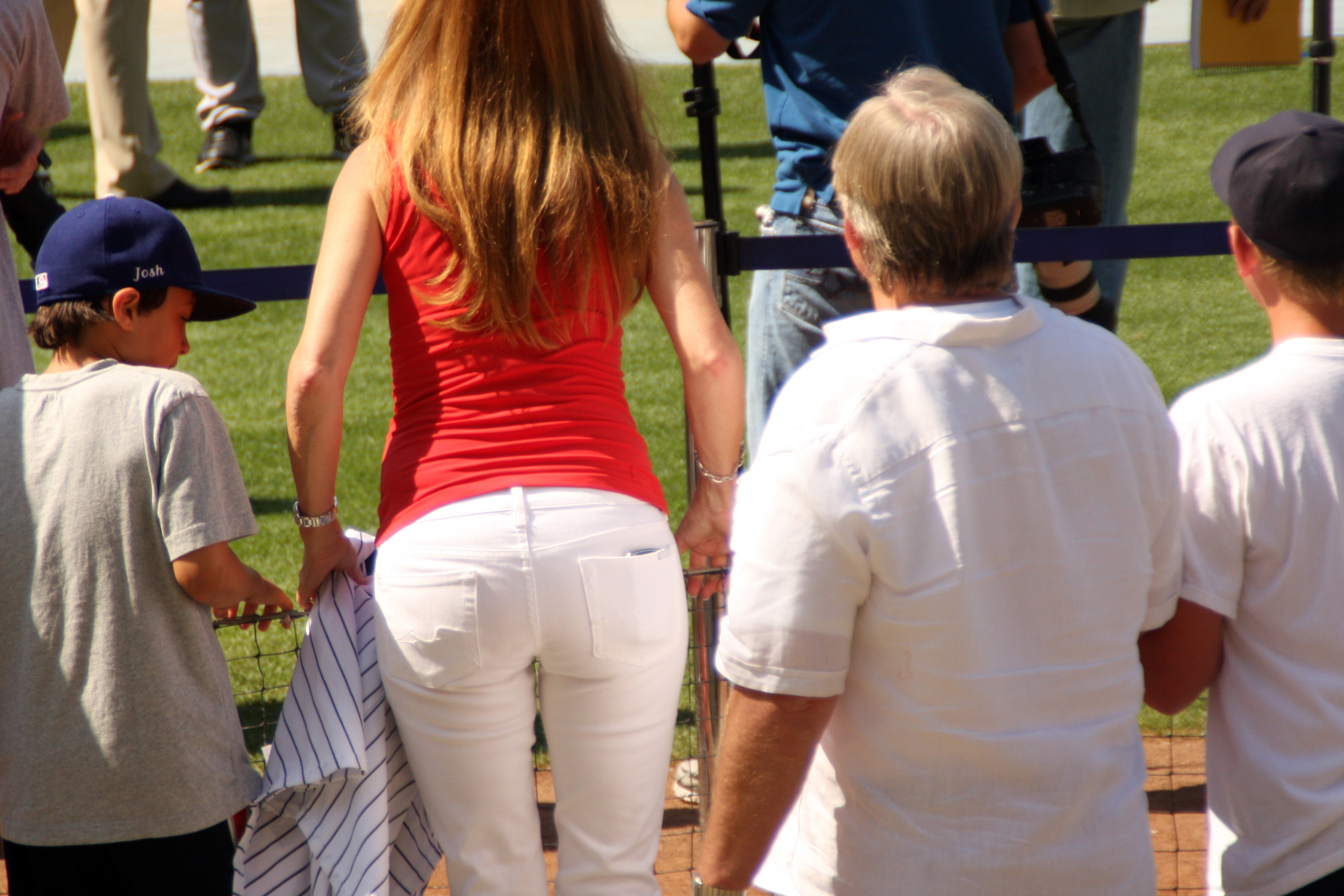In this square outdoor photograph, we see a group of onlookers from behind, focusing their attention on an event occurring on a green field. The central figure is a woman with long, reddish hair, dressed in white pants and a sleeveless red shirt, her left hand holding a black and white striped shirt, adorned with bracelets on both wrists. Next to her stands a young boy in a blue cap, gray shirt, and dark pants. Behind them is a slightly older, chubby man with graying hair, dressed in a white polo shirt. The scene is bustling with activity; numerous people, including a figure in a blue shirt, likely a golfer, and others in khaki pants and black shoes, are scattered across the grassy area on the other side of a barrier from the onlookers. The background is minimal, emphasizing the green expanse and the crowd gathered, possibly hinting at a golf event.